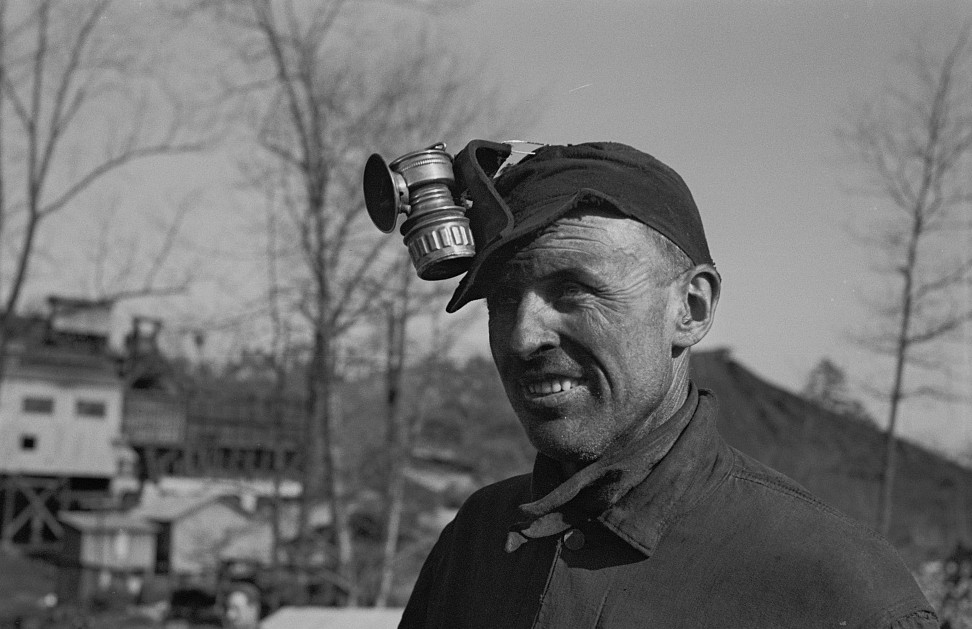This black-and-white photograph captures a weathered, elderly Caucasian man, primarily depicted from the shoulders up. The man, who appears to be a miner, has a face marked by deep wrinkles and a layer of grime, suggesting he has just finished working. He wears a black jacket buttoned up to his neck and a hat adorned with an old-fashioned headlamp. This headlamp has a large metal base and a small screen or globe at the front. His mouth is slightly open, revealing his top teeth, and he gazes to the left with a faint smile.

The blurred background features a composition of leafless trees—four in total—that stretch upward. On the left side of the image, there are several buildings, likely part of a factory or mining facility. These structures vary in size and some stand elevated on stilts. To the right, a large elevation, possibly a hill, can be seen. The overall scene exudes an industrial, rugged atmosphere, aligning seamlessly with the man's appearance and attire.